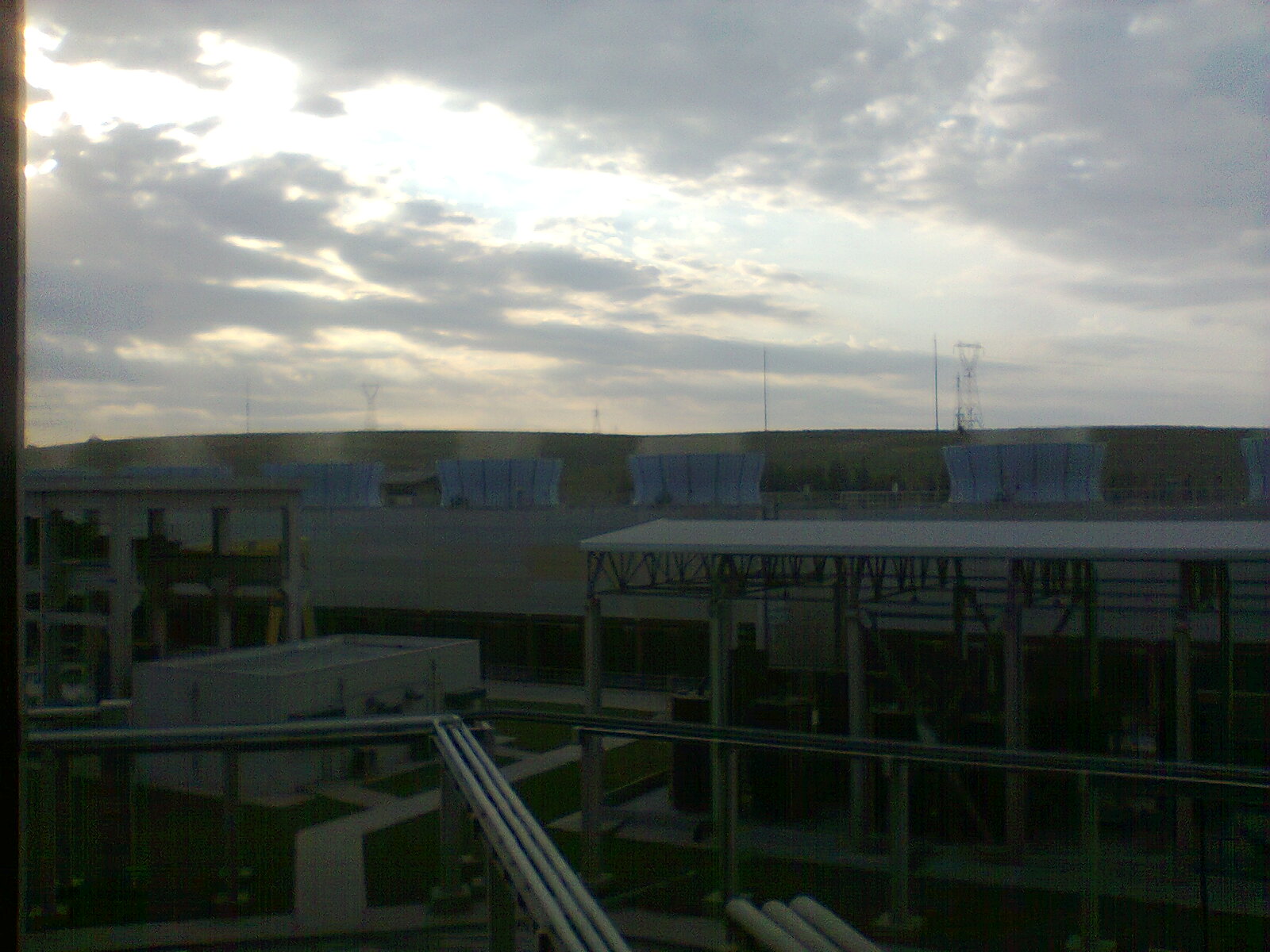The photograph captures an outdoor scene, likely taken through a window either in the early morning, late afternoon, or on a very overcast day. The sky is mostly cloudy with some glimpses of blue, and it appears quite bright on the left side. Below the sky, an industrial landscape unfolds, dominated by a construction site featuring a white building on the left side, surrounded by metal rods. Various white pipes are seen running parallel in the lower left quadrant, alongside a rectangular structure and an overhang housing materials or machinery in the lower right half. Distinctive cooling towers and chimneys or smokestacks are prominently positioned along the center of the image. Beyond these structures, green hills and power lines, including a large cable tower, stretch into the background, contributing to the complex layers of industrial and natural elements in the scene. The ground is covered in grass with a walkway cutting through it, adding a touch of greenery to an otherwise industrial setting.